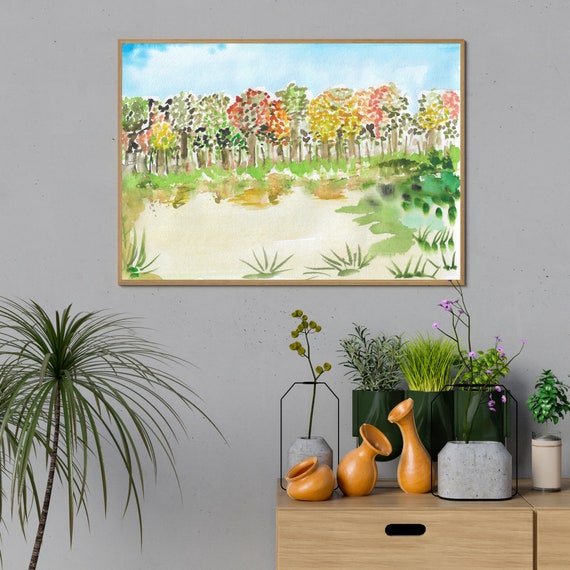The photograph showcases the interior of a room with a prominent painting as its central focal point, mounted on a gray wall. The painting, enclosed in a thin brown frame, vividly depicts multicolored trees against a blue sky scattered with clouds, suggesting a possible watercolor technique. The trees, rendered in an abstract manner with short, almost brush-tip-like strokes, encompass shades of green, brown, yellow, orange, and red. The scene includes water beneath the trees, reflecting the lush foliage above.

In the foreground, a small, office palm plant stands to the left of the painting. To the right, a light wooden desk—blonde in hue—hosts an array of vibrant plants. This wooden desk includes a drawer indicated by a visible handle. The plants vary, with most being shades of green, while one features striking purple flowers. The arrangement also consists of three brownish clay vases with large openings, enhancing the artistic atmosphere of the space. The greenery appears well-matched to the decor, blending naturally with the aesthetic of the room.